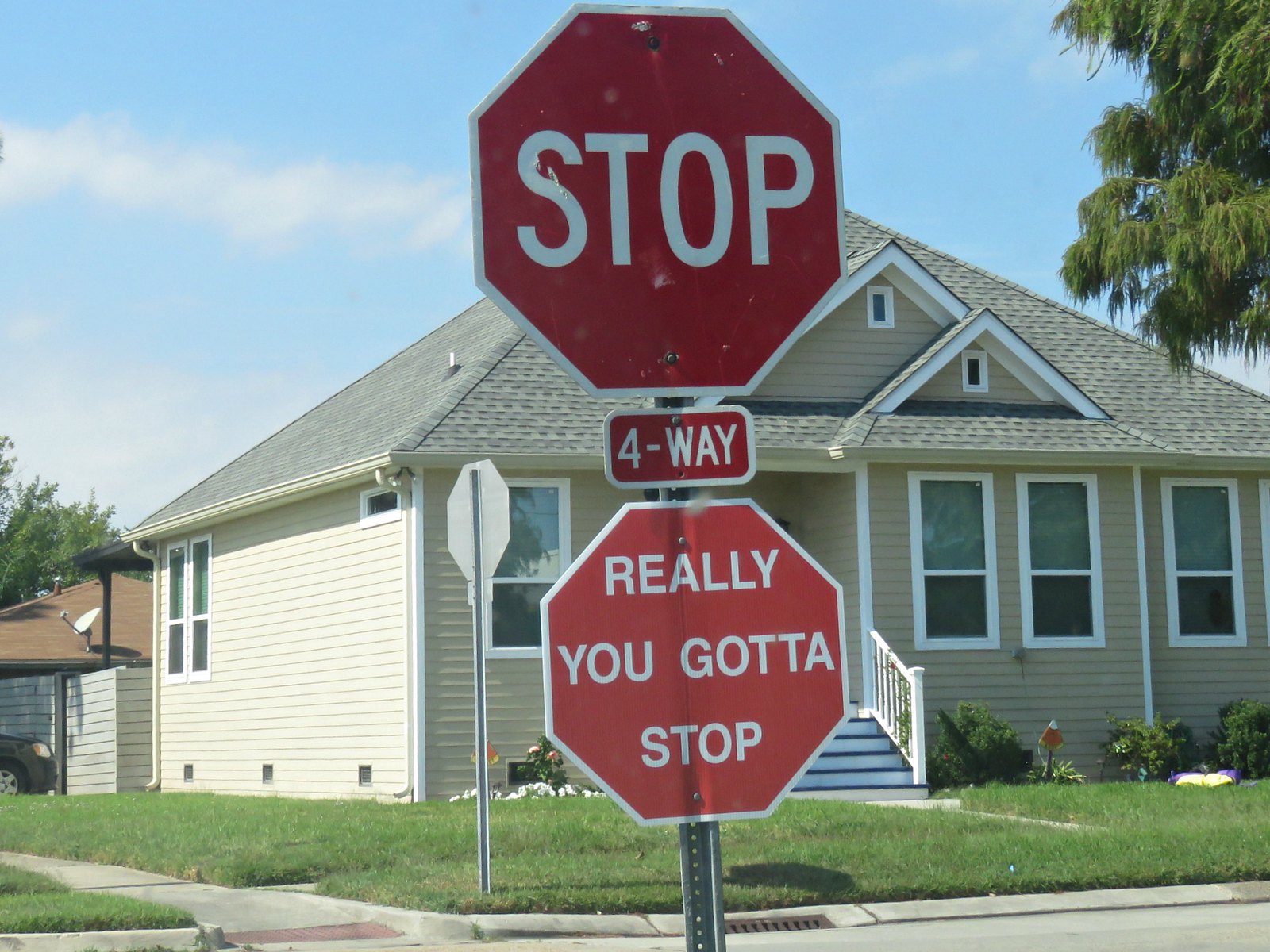This photograph captures a residential street corner on a clear day with a blue sky and white clouds. Prominently featured in the foreground is a standard red and white stop sign atop a pole, accompanied by a smaller sign reading "4-WAY" directly below it. Below this is another red, stop-sign-shaped placard with a playful inscription in white letters: "REALLY, YOU GOTTA STOP," hinting at a community addition. In the background stands a beige bungalow-style house with blue steps leading to its front entrance. The house is surrounded by a green, grassy lawn and bordered by a tan fence. A car is parked alongside the house, and a tree extends into the right side of the scene. Sidewalks frame the intersection, where a visible grate is noted on the street in front of the house, adding to the residential ambiance.